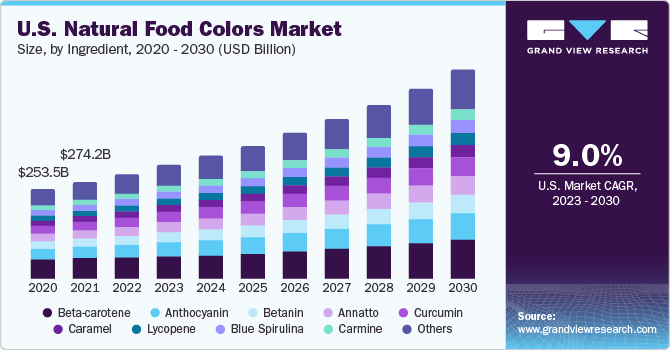This detailed infographic in landscape orientation illustrates the U.S. natural food colors market from 2020 to 2030, highlighting market size by ingredient (in USD billion). Dominating the left three-quarters of the image is a bar chart, with bars increasing in height from left to right, spanning 11 increments. The first bar represents the year 2020, and the last one represents 2030. Each bar is segmented and color-coded to denote various natural ingredients: beta carotene, anthocyanin, betanine, annatto, curcumin, caramel, lycopene, blue spirulina, carmine, and others. On the top left corner, bold black text reads "U.S. Natural Food Colors Market," followed by smaller text detailing the time frame and measurement unit. 

On the right side of the image is a dark blue vertical rectangle displaying key metrics in white text, including a 9.0% CAGR for the U.S. market from 2023 to 2030. The letter V in "CAGR" is styled as an upside-down turquoise triangle. At the top of this section, a white and blue "Grandview Research" logo is prominently displayed, and the source of the data, www.grandviewresearch.com, is noted at the bottom in white text. The comprehensive layout and color-coding effectively communicate the growth and composition of the market over the decade.